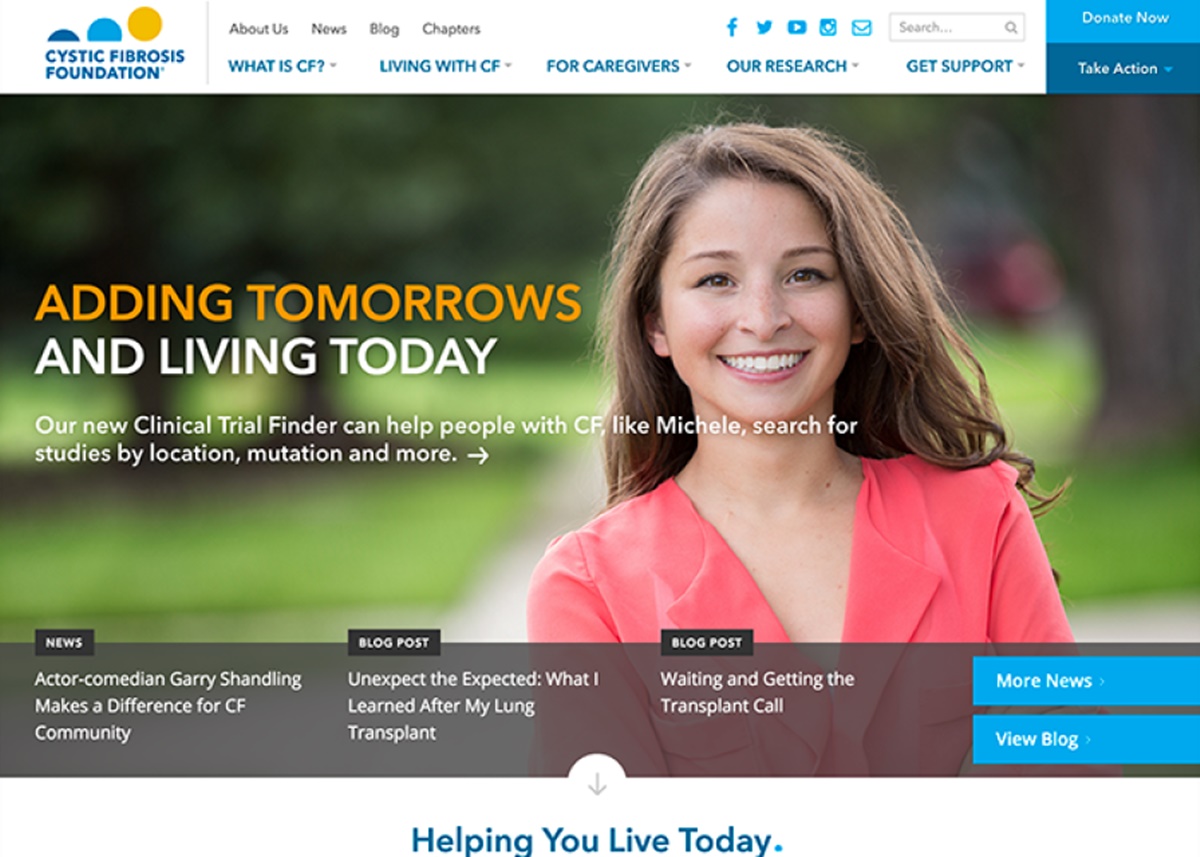The image showcases a website layout that is approximately 30-50% wider than it is tall, though the bottom edge is undefined, blending into a white background that occupies the lower 10-15% of the image. At the top, a header area is prominently displayed, indicating that this is a website. In the upper left corner, "Cystic Fibrosis Foundation" is written in blue text, with three colored circles (dark blue, light blue, and yellow) arranged like a staircase starting above the text. Only 20% of the first circle is visible, followed by 80% of the second circle, and the entirety of the third circle.

To the right of the foundation's name, four black-text menu options are listed: "About Us" and "Blogger Chapters," followed by a section in larger font that serves as the main site navigation. This section includes menu options in light blue: "What is CF," "Living with CF," "For Caregivers," "Our Research," and "Get Support." Above "Get Support" is a search bar, and above "Our Research" are various social media icons. Additionally, to the right of these navigation options, there are two call-to-action buttons: a light blue box with the text "Donate Now" and a dark blue box with the text "Take Action."

Dominating the lower half of the image is the main banner, featuring a young woman smiling warmly at the viewer, creating an inviting atmosphere for the website's visitors.